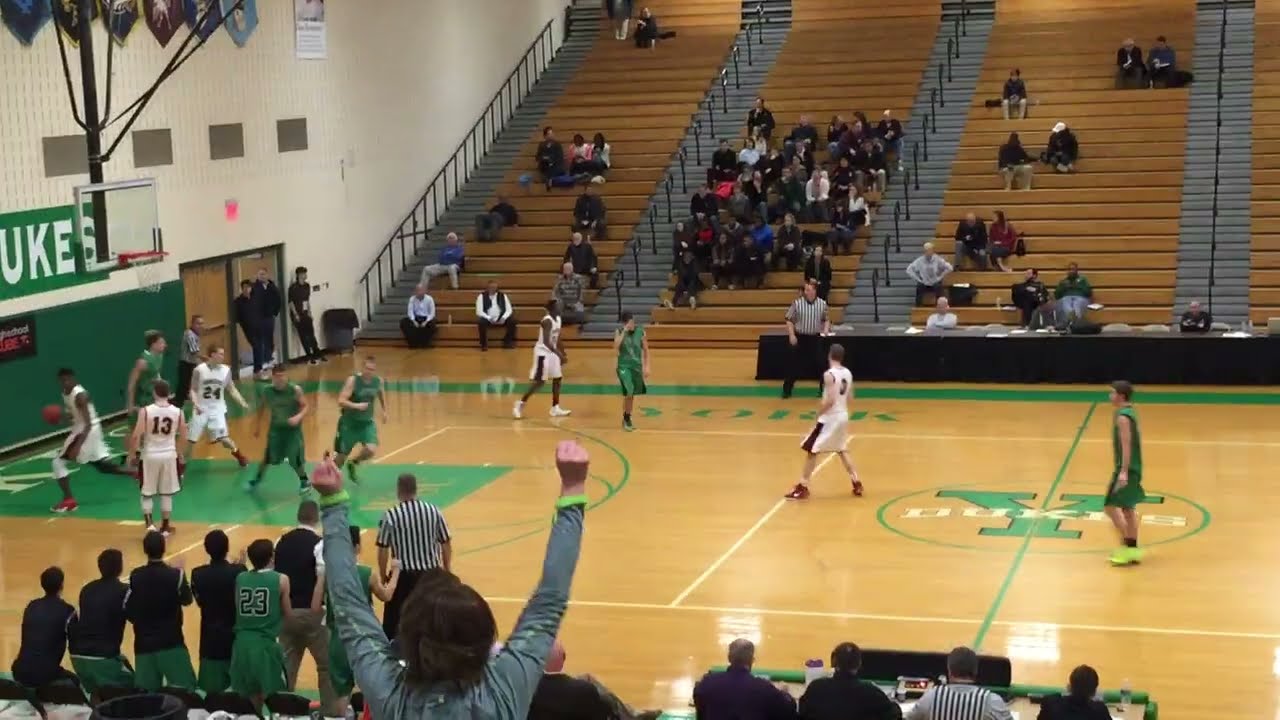This image captures the vibrant scene of an indoor high school or college basketball game in a gymnasium. The gymnasium floor is light brown, featuring a prominent green 'Y' symbol at center court, with 'Dukes' inscribed in white lettering above it. The two teams in action are the green team and the white team. On the court, a player in a white uniform with the number 13 is facing away, while another white-uniformed player with the number 24 is facing forward. The green team has players wearing predominantly black shirts and green shorts, with one player distinctly noticeable in a green jersey marked with the number 23.

Spectators populate the scene as well; notably, a woman in gray, positioned in the foreground on the left, is raising her arms in triumph with her elbows straight. Behind her, on the right side of the image, the audience sits in light brown bleachers interspersed throughout, though primarily concentrated in the center. There's a table with officials or statisticians near the court, with a referee stationed in front and another near the basketball net on the left side.

Visible also are the gym's white walls adorned with high banners and the ceiling extending up to the stadium rafters. The atmosphere is lively, with people on the bench standing excitedly, reflecting the competitive spirit of the game.